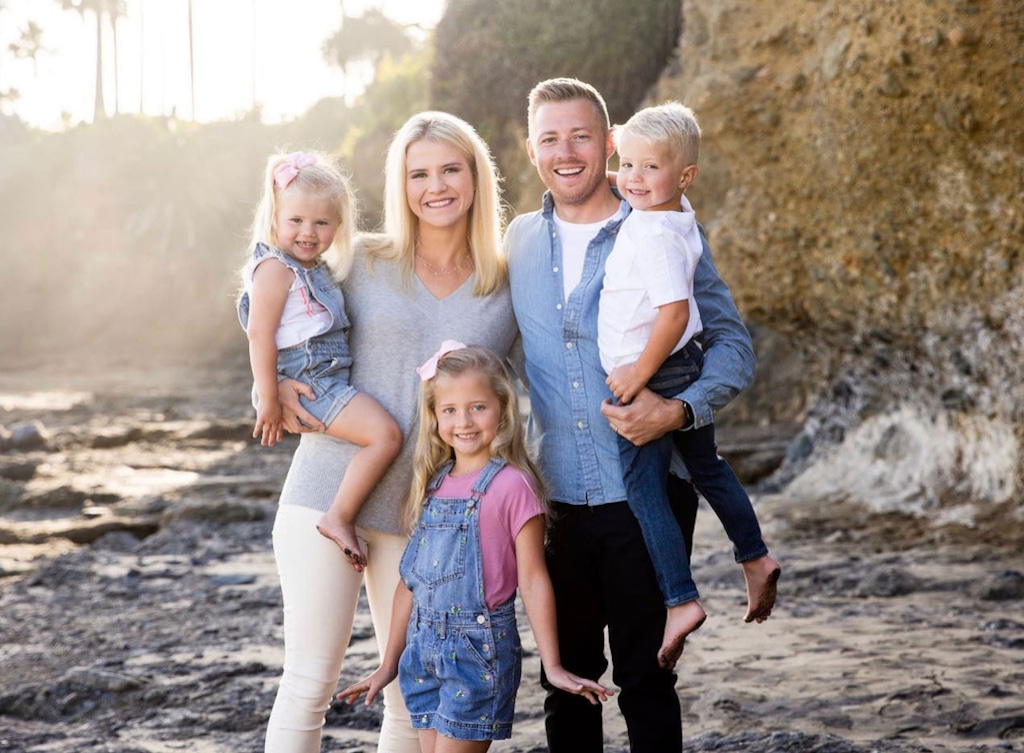A professional family portrait captures a tender moment on a rocky beach, with a picturesque backdrop of trees, water, and blurred foliage. The fair-haired mother, donning a grey V-neck shirt and tan pants, holds the youngest daughter, a blonde girl dressed in denim dungarees shorts and a white T-shirt adorned with a pink illustration, who is barefoot with dirty feet and a pink bow in her hair. Beside them stands the father, wearing a white T-shirt under a blue button-up shirt paired with black pants. He cradles their fair-haired son, clad in a white shirt and dark blue jeans, also barefoot with muddy feet. Between the couple stands their eldest daughter, around five to seven years old, in a pink T-shirt and blue denim dungaree shorts, matching her sister's pink bow. The scene is set against grey, rough ground with an element of a stone wall or mountains in the distance, further enhanced by the light filtering through, adding warmth to this serene, beachy family setting.